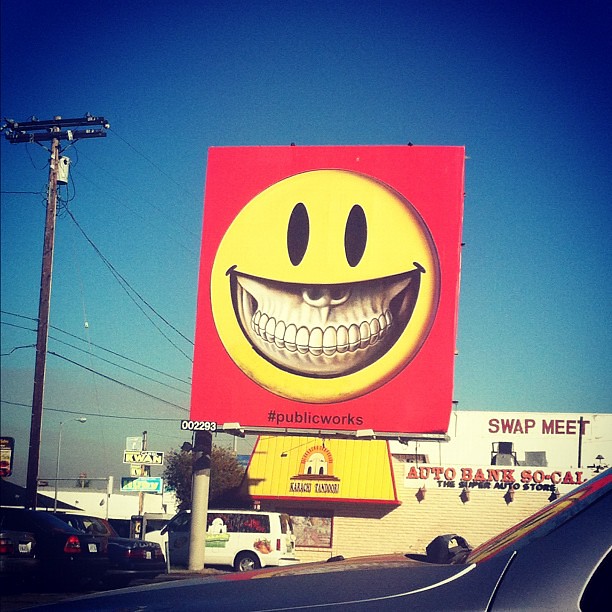This photograph, taken in the late evening when the sky is a deeper, darker hue than daylight, captures a parking lot scene. In the foreground, several vehicles are parked, including a white van and darker-colored cars adjacent to it. Dominating the background is the side of a building adorned with various signs, including "Swapmeet" and "Auto Bank SoCal." A yellow awning promotes "Karachi Tandoori," an Indian restaurant. In front of the building stands a cement pole supporting a prominent red billboard. This billboard features a large, classic yellow smiley face with an eerie twist: the grin reveals the skeletal teeth and nasal cavity of a skull. Below this striking image, the hashtag "#publicworks" is visible. To the left, a telephone pole, rising just about even with the top of the billboard, highlights the structure's height. The scene is further detailed with clear skies and visible electrical poles and wires, contributing to the urban setting.